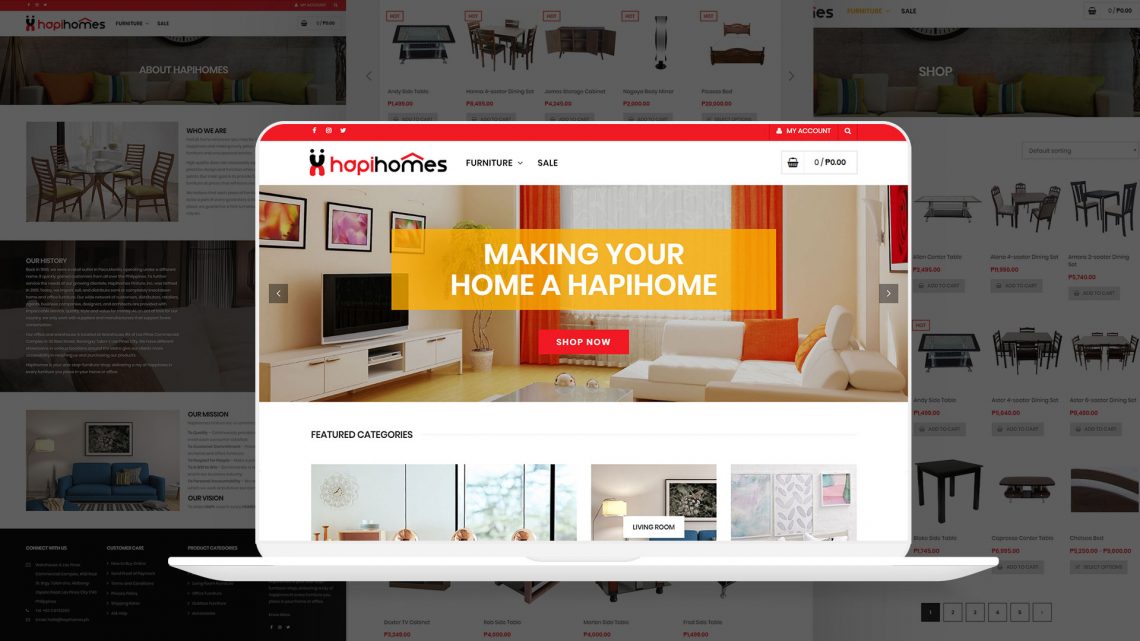A detailed advertisement for Happy Homes is prominently displayed as a pop-up on a mobile website version. In the background, the Happy Homes logo is visible, reinforcing the brand. The main page showcases a cozy living room setup featuring a stylish couch adorned with vibrant orange cushions, positioned across from a television on an elegant entertainment center. The decor includes various pictures on the back wall, enhancing the inviting atmosphere.

The tagline, "Making your home a happy home," is artistically crafted with the word "happy" spelled as "h-a-p-i" in orange letters outlined in white. Additionally, a red square with white lettering urges viewers to "Shop Now," adding a sense of urgency and enticing immediate action.

Below the main banner, the website highlights different featured categories, such as Living Room, Bathroom, and more. The majority of the background imagery depicts an array of furniture, including beds, tables, chairs, and a distinctive big blue couch, illustrating the diverse range of household goods available for purchase. This engaging and visually rich web page aims to motivate customers to explore and buy quality furniture and home accessories to enhance their living spaces.